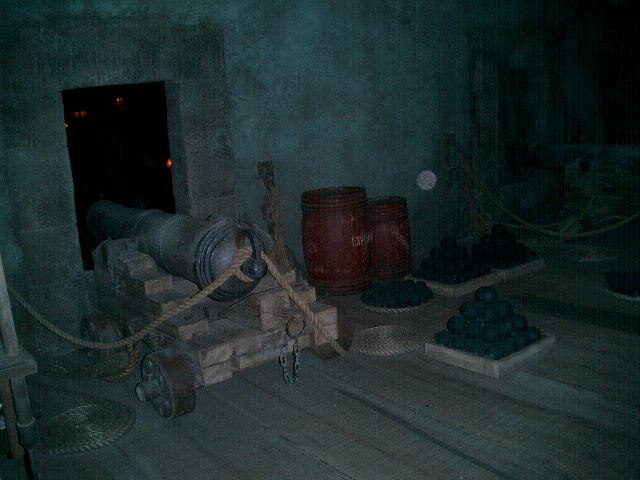This photograph showcases an indoor museum display, possibly in a war museum or historical bunker. The room, with its dark concrete walls and wide wooden plank floors, features a prominent antique cannon positioned on a sturdy wooden cart with metal wheels, pointing out through a cut-out window in the wall. There are ropes coiled at the back of the cannon, extending towards the wall and lying on the ground. On the left side of the image, the cannon is surrounded by stacked cannonballs arranged in pyramid shapes, and there are two wooden barrels placed against the wall. The barrels, one slightly taller than the other, are similar in height to the cannon and are labeled "explosives." The overall atmosphere is enhanced by the dusty, aged look of the photograph, underscoring the historical significance and antique nature of the display.